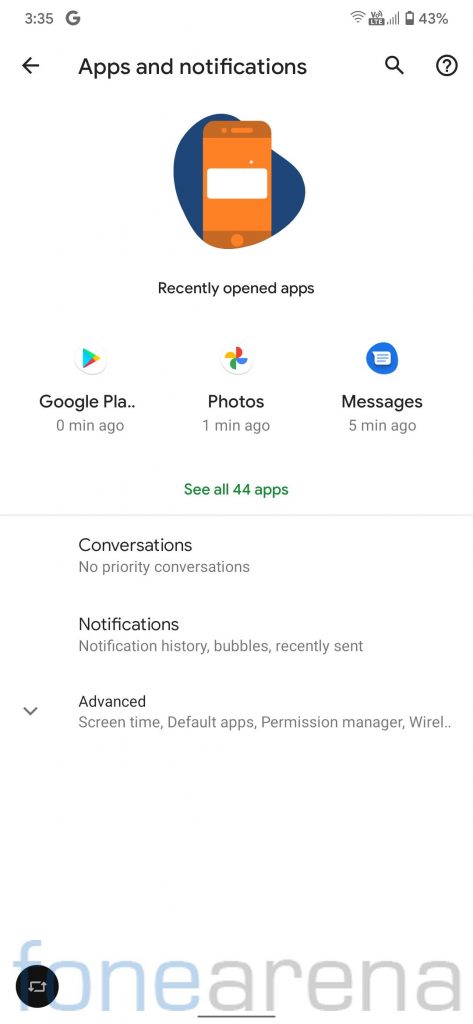This image appears to be a screenshot taken from a smartphone, which is indicated by the status bar at the top displaying "3:35 PM", Wi-Fi signal strength, battery life at 43%, and network bars. 

The screenshot captures a settings page titled "Apps & notifications". Below the title, there is a section similar in shape to a painter’s easel, containing a red box with a white rectangle in the middle. This section lists "Recently opened apps":

1. Google Play – zero minutes ago
2. Photos – one minute ago
3. Messages – five minutes ago

There is a link to "See all 44 apps" to view the complete list.

Following that, there's a section labeled "Conversations", stating "No priority conversations".

Next, the "Notifications" section includes subcategories:
- "Notification history"
- "Bubbles"
- "Recently sent"

Lower down, the "Advanced" settings feature:
- "Screen time"
- "Default apps"
- "Permission manager"

Below this, the screen appears to cut off with the partial word "wire..."

At the very bottom, there is a reference to a webpage from "Phone Arena" (stylized as F-O-N-E-A-R-E-N-A), with the letters A-R underlined. Above the letters "F" and "O", there is a black oval icon containing arrows pointing up and down, signifying share options, such as sharing the webpage or a screenshot with others.